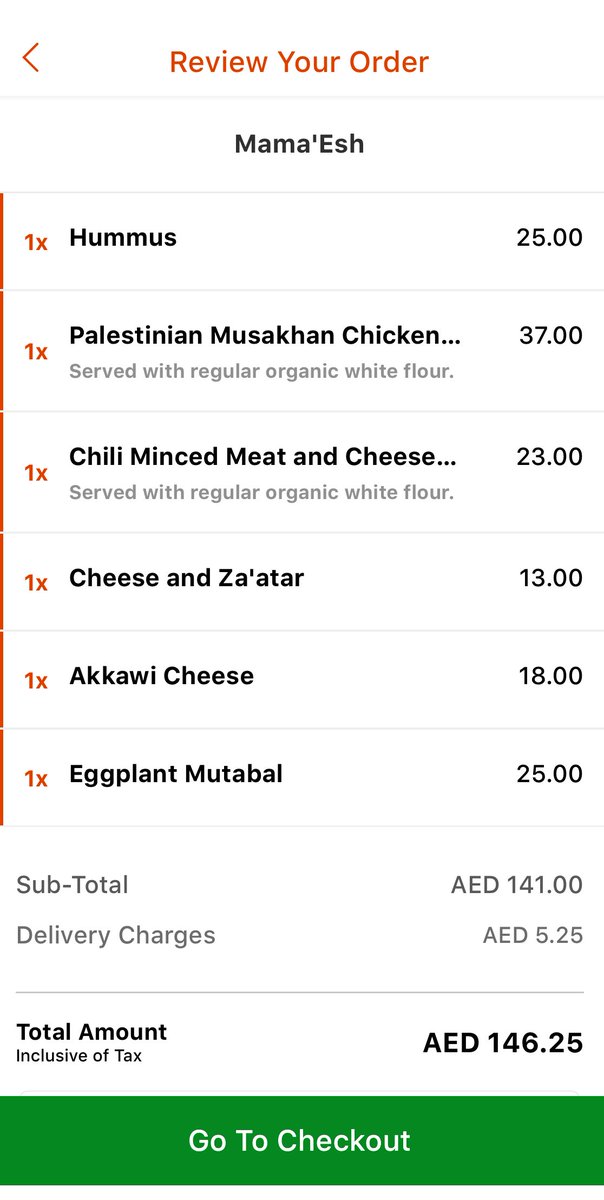The image features an online order review screen for the restaurant "Mama Ish." At the top, an orange banner with an arrow pointing left reads "Review Your Order." Below this banner, the restaurant's name, "Mama Ish," is prominently displayed in black font.

The order details include several items:
- Palestinian Muscat Canned Chicken: AED 37.00
- Chili Mince Meat and Cheese served with Regular Organic White Flour: AED 23.00
- Cheese and Za'atar: AED 13.00
- Akawi Cheese: AED 18.00
- Eggplant Mutabal: AED 25.00

The subtotal for the items amounts to AED 116.00. However, there's an additional delivery charge of AED 25.00, bringing the total cost to AED 146.25, inclusive of tax. 

At the bottom, a thick green bar with white text reads "Go to Checkout," directing users to proceed to the payment and delivery setup.